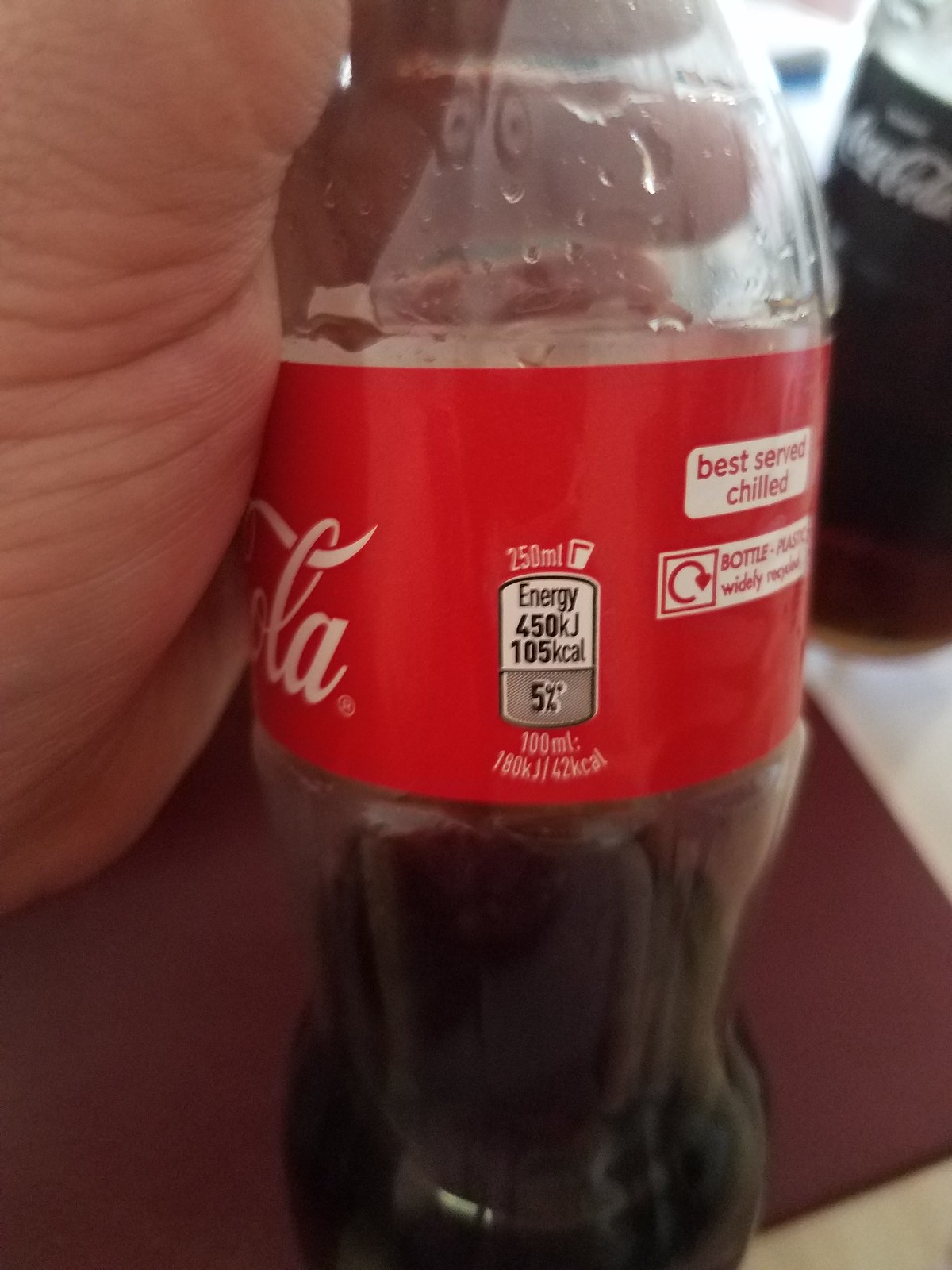The image depicts a partially empty plastic Coca-Cola bottle, with a small amount of dark liquid, likely Coke, visible at the bottom. The transparent plastic reveals carbonation bubbles clinging to the innermost edges, indicative of the effervescent nature of the beverage. A bright red label wraps around the bottle, a distinctive color associated with the Coca-Cola brand. The prominent logo "Coca-Cola" is partly visible, showing the letters "O-L-A," as the bottle is held by a light-skinned hand. The front of the label displays the volume "250 milliliters" in bold white characters. Additionally, two white informational boxes are embedded within the red label. One box, with red text, advises that the drink is "Best Served Chilled," while the other features a recycling icon, a partial circle with an arrow pointing to the right and downward. The bottle is photographed against a brown surface that rests on a lighter-colored background.